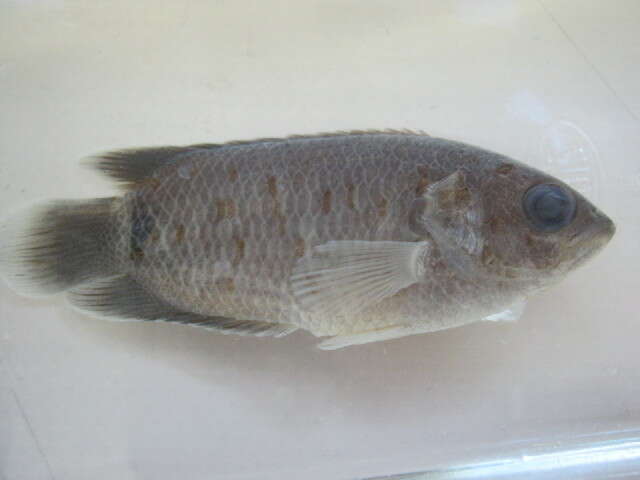The image features a gray fish, likely a 'Tenopoma kingsleyae,' displayed on a white dish or examination paper within a store counter for sale. The fish, which isn't very large, lies on its side with its tail pointing to the left and its head facing the right. Its body is predominantly gray with specks of brown and black, giving an impression of spots. The fish has a large, round, bluish-gray eye and a translucent white fin towards the bottom right. The tail, which has a white tip and darkens where it meets the body, accentuates the dark hues of the fish's body. The presentation evokes a sense of stillness and finality, contrasting with the fish's once lively existence in its native waters from regions like Senegal, the Democratic Republic of the Congo, and the Congo River basins.